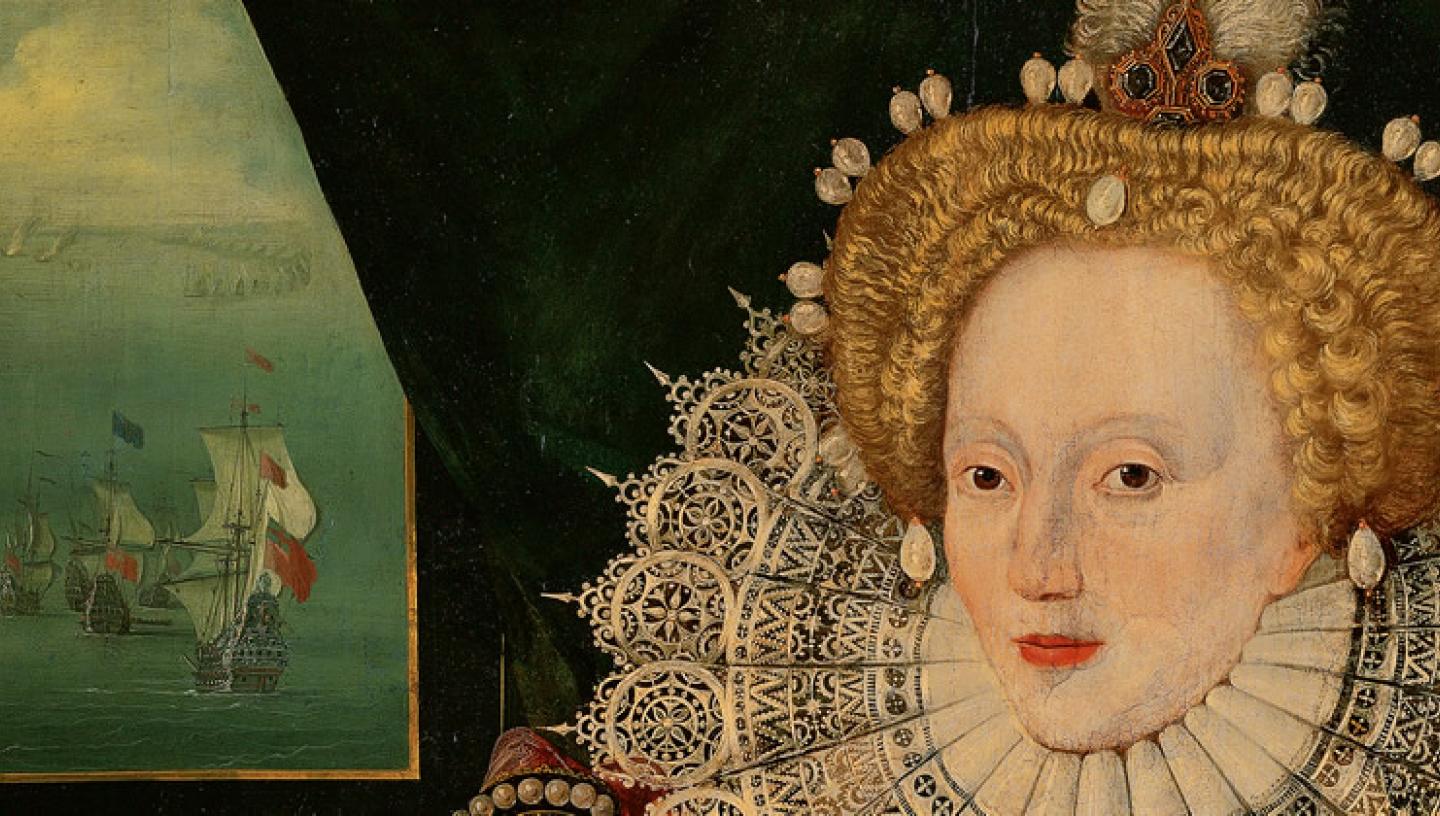This image is a detailed, cropped section of a Renaissance-era oil painting, approximately five inches wide and three inches tall. On the right half, it prominently features a striking portrait of Queen Elizabeth I. Her oval face is powdered white, enhancing her thin, barely visible eyebrows and expressive brown eyes. She has slightly rosy cheeks and bold reddish-orange lips. Her hair, a vibrant orange, is styled in tight curls that frame her head in a halo-like shape. Adorned with teardrop-shaped pearls and a headdress that includes a black brooch and a combination of red and white feathers, her coiffure is both elaborate and regal. Perched atop her head is a diminutive crown with feathers protruding from it.

Around her neck, Elizabeth wears an intricate, wide ruffled collar, adding to her imposing presence. The background on her right features a dark, almost black deep green hue, giving prominence to her figure. To the left of her and comprising the left half of the image, there is a maritime scene, likely viewed through a window or depicted as a painting within the painting, showing a fleet of sailing ships on a calm ocean. The weather appears fair with perhaps a suggestion of exploration or naval importance. This composition, rich in historical and decorative elements, captures the regal essence of Queen Elizabeth I against the backdrop of an era defined by sea voyages and nautical discoveries.